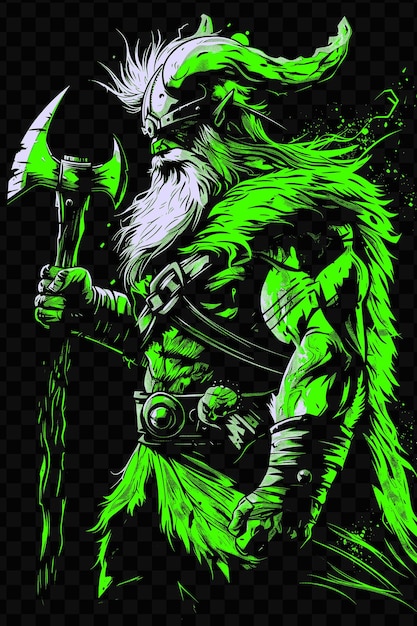This detailed digital illustration presents a fantasy-themed depiction of a Viking-like figure, set against a pitch-black background. The artwork primarily utilizes three colors: black, white, and a striking neon kelly green. The character, rendered in a profile view, is shrouded in mystery with no visible facial features but is distinguished by his long, white hair and matching beard. He is adorned with a Viking helmet, accentuated by green highlights and sporting horns. Green feathers or perhaps fur embellishments cascade from the front of his helmet to the back. 

The Viking's attire is detailed with a fur-lined vest, multiple leather belts—one cinched around his waist and another slung diagonally from shoulder to waist—and heavy gloves, all finely highlighted in neon green. His right hand grips a formidable double-edged axe, its sharp, pointed blade illuminated with the same vivid green hue. The white lines contrast sharply against the dark backdrop, while the bright green elements highlight significant aspects such as the horn, hair, fur accents, arms, and parts of the axe, adding a dynamic glow to the otherwise monochromatic scheme. This clear and well-lit image captures the essence of a mythical warrior poised in a moment of intensity.